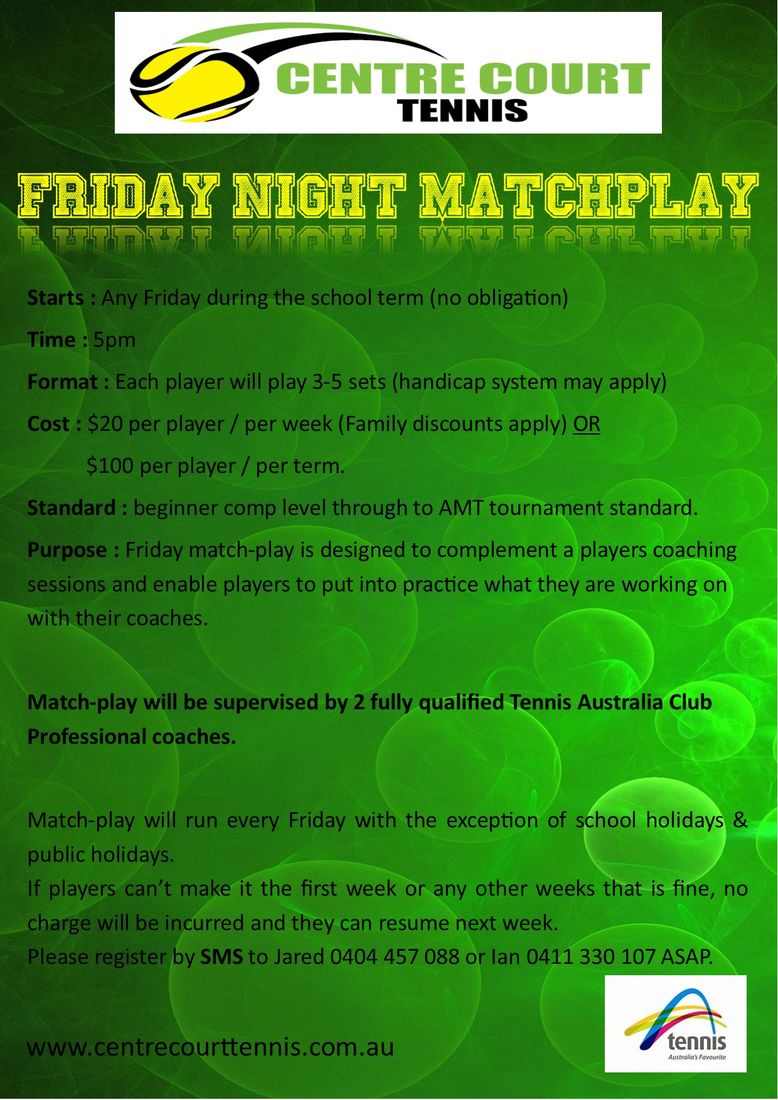The image is a promotional poster for a tennis event held by Century Center Court, with a vivid lime green background featuring a pattern of green tennis balls. Central in the image, a white rectangular box contains the event title, with "Century Center Court" in light green text and "Tennis" in black text. A yellow tennis ball icon is situated to the left. Below this, in prominent yellow text, it reads "Friday Night Match Play."

The detailed event information is given in various colored texts. The text outlines that the match play starts at 5 p.m. any Friday during the school term, with no obligation to attend every week. The format indicates that each player will play 3-5 sets, potentially under a handicap system. Costs are specified as $20 per player per week, with family discounts available, or $100 per player per term. Additional content emphasizes that Friday match play aims to complement coaching sessions, allowing players to put their training into practice under the supervision of two fully qualified Tennis Australia club professional coaches. Matches will not be held during school and public holidays, and there is flexibility for players who cannot attend every week without incurring charges.

Registration details include contact information for Jared (0404457088) or Ian (0411330107) and a website for further information: www.centercourttennis.com.au.